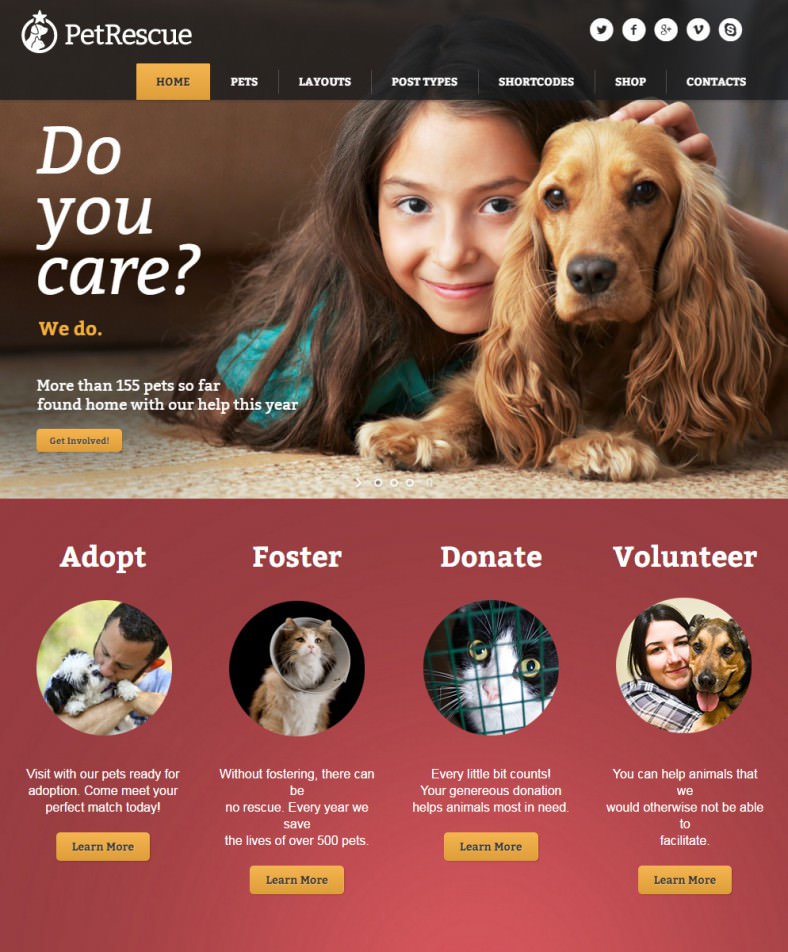This image is an advertisement for a pet rescue organization. At the very top, there is a black banner. On the left side of the banner, "Pet Rescue" is written alongside a white icon featuring a cat and dog under a star. On the right side of the banner, there are links to the organization's social media pages, including Twitter, Facebook, Google Plus, Vimeo, and Skype.

Below this banner, the top of the page features navigation tabs labeled Home, Pets, Layouts, Post Types, Short Codes, Shop, and Contacts. The Home tab is highlighted in yellow, indicating the current page view.

Prominently displayed at the top of the page is an image of a girl smiling warmly as she pets a golden retriever puppy. The girl is wearing a blue shirt. Superimposed on this image is the text, "Do you care? We do. More than 155 pets so far have found homes with our help this year." Beneath this text is a yellow button with the phrase "Get Involved."

Below this section is a deep, muted red banner featuring four different images. Each image is accompanied by captions and a yellow "Learn More" button. The images and their corresponding captions are:
1. Adopt – Featuring a picture of a dog.
2. Foster – Featuring a picture of a cat.
3. Donate – Featuring another animal image.
4. Volunteer – Featuring yet another animal image.

This advertisement effectively conveys the mission of the pet rescue organization and provides clear options for how individuals can get involved, whether through adoption, fostering, donating, or volunteering.